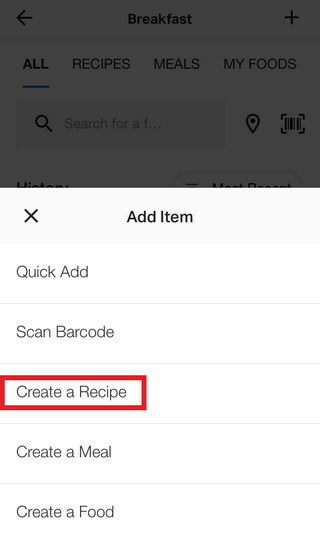The image is set against a crisp white background and features a series of menu options related to breakfast and meal management.

At the top, there is a grey box that prominently highlights the word "BREAKFAST". This grey box includes a left-facing arrow icon on its left side and a plus sign icon on its right side.

Directly below this, the menu is presented from left to right, starting with "ALL" which is distinguished by a blue underline to indicate it is the selected option. Following "ALL", the other menu choices are labeled as "RECIPES", "MEALS", and "MY FOODS".

Underneath the menu options, a search box is situated, with a magnifying glass icon on the left and a pin icon on the right, allowing users to search for specific items.

Beneath the search box, in bold grey text, is the phrase "Add Item". Following this text, there are additional menu options displayed in light grey text. These options include "Quick Add", "Scan Barcode", and "Create a Recipe". "Create a Recipe" stands out with a red border highlighting it. Finally, the menu continues with "Create a Meal" and "Create a Food".

Overall, the image clearly outlines a structured interface for managing breakfast-related items and activities.